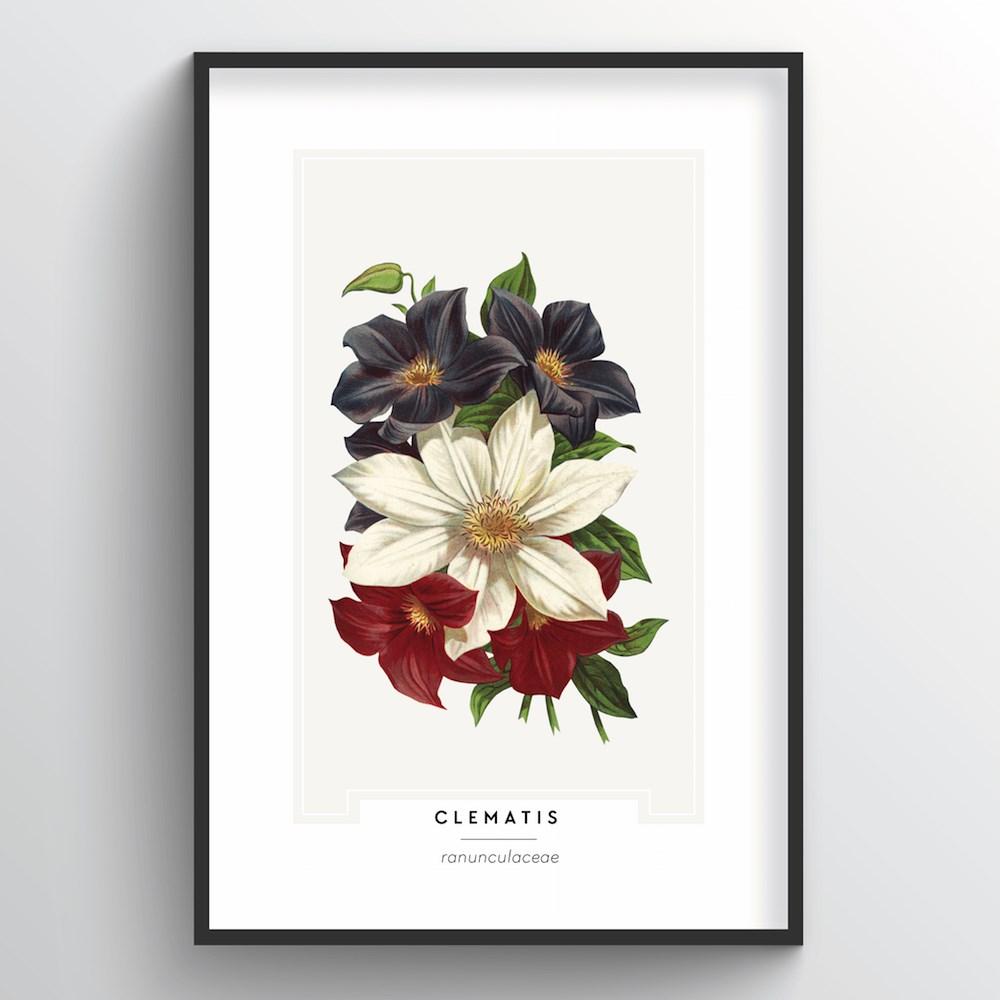The image is a digitally rendered product photograph intended for commercial use, such as in online shops or catalogs. It features a rectangular poster encased in a thin, black frame. The frame is set against a flat, light gray background, giving the impression that it is hanging on a wall. The poster itself has a sizeable white border surrounding the main artwork. At the bottom of this border, in black text, it reads "Clematis," followed by a horizontal line and the text "Ranunculaceae" in smaller gray print. The central artwork within the poster consists of a very light pale gray, almost white, background. The composition showcases a bouquet of flowers: a large white flower with elliptical petals at the center, flanked by two smaller red flowers beneath it and two black flowers above. The flowers all feature gold-colored centers, surrounded by green leaves. Overall, the image emphasizes a clean, minimalistic aesthetic, with a clear, synthetic quality indicative of digital editing.